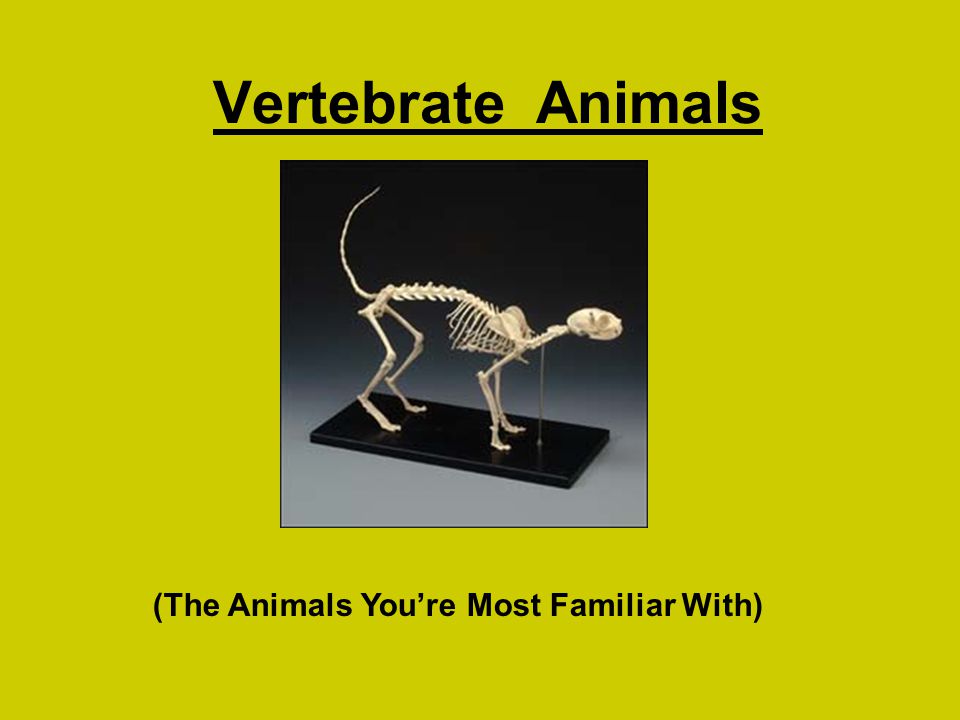The image depicts a detailed model of a vertebrate animal skeleton, positioned centrally within a square frame. The skeleton, set on a rectangular black platform, features the skull facing to the right and a slender tail raised to the left. The animal has four legs, with the front limbs and bent hind limbs resting on the platform. The background of the square is black at the top, transitioning to light gray at the bottom. Encasing this scene is a mustard yellow (or yellowish green) background. At the top of the image, centered in bold black text and underlined, the title reads "Vertebrate Animals." Below this, in parentheses, it states, "The animals you are most familiar with."